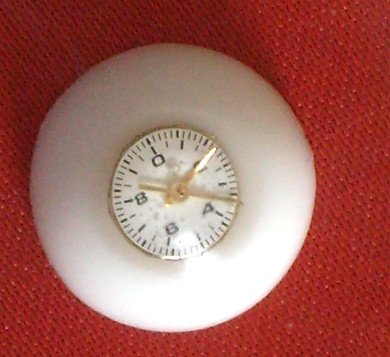This image showcases a unique, small-sized clock with an unconventional design. The clock features a white outer casing and a gold center where the clock hands are mounted. The hour and minute hands are also gold, which harmonizes with the central part of the clock. Unlike standard clocks, this one has numbers arranged in an unusual sequence: 0, 2, 4, 6, and 8, written in black. The entire clock is set against a richly textured red fabric background, which adds a vivid contrast and highlights the elegant colors of the clock itself. The material's weave is clearly visible, adding an extra layer of detail to the overall composition. The image’s color scheme is predominantly red, white, gold, and black. It remains unclear whether this clock is being showcased for sale or merely as an example of an intriguing design.